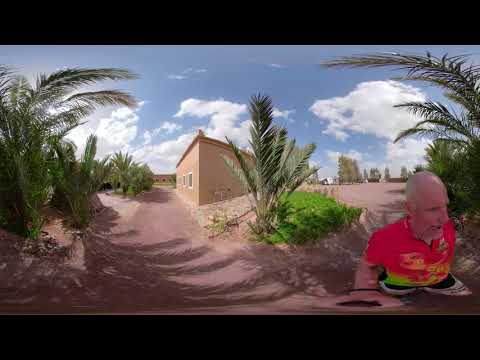The image captures a serene outdoor scene featuring a tan, rectangular building with white windows set against a backdrop of a clear blue sky with soft, white clouds. The foreground is dominated by reddish-brown soil, suggesting a desert-like environment, and adorned with tropical-looking plants, possibly ferns or palm trees, strategically positioned on the left, middle, and right sides of the photograph. These plants cast gentle shadows towards the lower left. To the right of the house, a vivid green patch of grass provides a contrast to the surrounding arid landscape. On the bottom right corner, a bald Caucasian man dressed in a bright red shirt is visible, gazing towards the right side of the image. He adds a human element to this tranquil, sunlit scene.